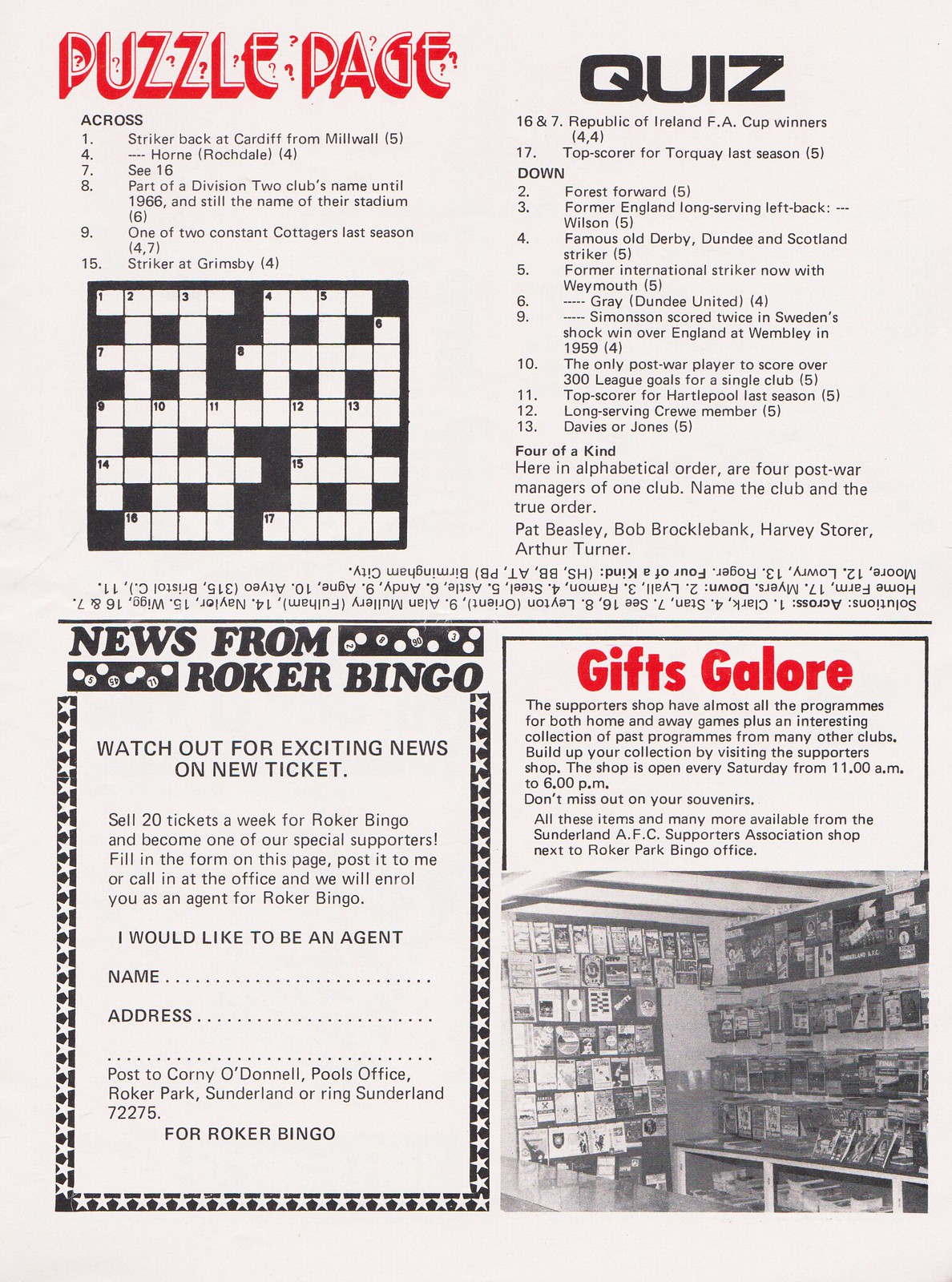The image appears to be a scan of a magazine or newspaper page with a light blue background, divided into four distinct sections. The top left section is labeled "Puzzle Page" in red font with a white border. This section features various clues numbered 1, 4, 7, 8, and 9, corresponding to a crossword puzzle located at the bottom of this block. The crossword puzzle is square and fairly simple, featuring a grid of empty squares.

The top right section is labeled "Quiz", also in red text, and includes several questions numbered 16, 17, 2, 3, 4, 5, 6, 9, 10, 11, 12, and 13, with a strong soccer theme, including specific trivia such as "Forrest Ford, former England long-serving left-back." Below this quiz section is a block labeled "4 of a kind," presenting additional clues for the crossword puzzle. The solutions to the crossword are printed upside down in small black text beneath these clues.

The bottom left section of the page features news from "Roker Bingo," with headlines such as "Watch out for exciting news on new tickets" and an offer to become an agent by selling 20 tickets a week. A form is included for potential agents to fill in their name, address, and contact details, encased in a black border adorned with white stars.

The bottom right section is titled "Gifts Galore" in red text. Following this title is a paragraph of descriptive text, as well as a black and white photograph of a shop displaying various products, possibly picture frames, though the details are small and unclear. The entire page has an off-white tone that adds to its vintage appearance.